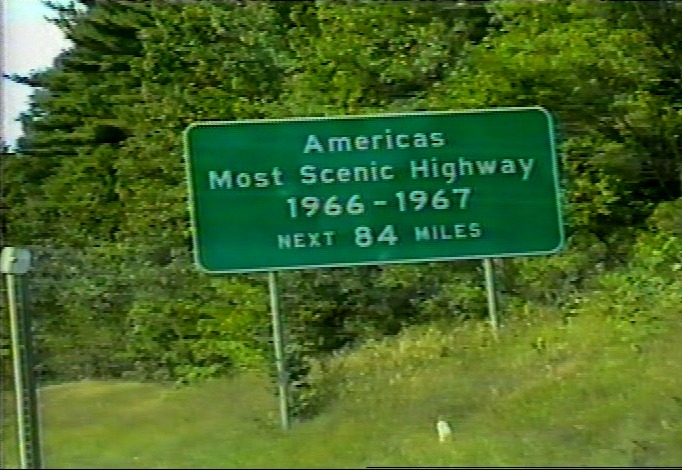The image features a roadside highway sign prominently displayed in a grassy area. The sign is rectangular, green, with white lettering and a white border, and it reads: "America's Most Scenic Highway, 1966 to 1967, Next 84 Miles." This sign is supported by two wooden poles, with the right pole slightly shorter due to a rising bank. In front of the sign is a stretch of green grass, with some low-growing bushes around the base of the poles. Behind the sign, a dense forest of both deciduous and fir trees, all lush and green, can be seen. The sky is partially visible in the upper left, showing a bit of blue with some white clouds. The image seems to be taken through a window, as there's a faint reflection visible. The overall scene is very green, with the sign standing out against the natural backdrop of trees and grass.